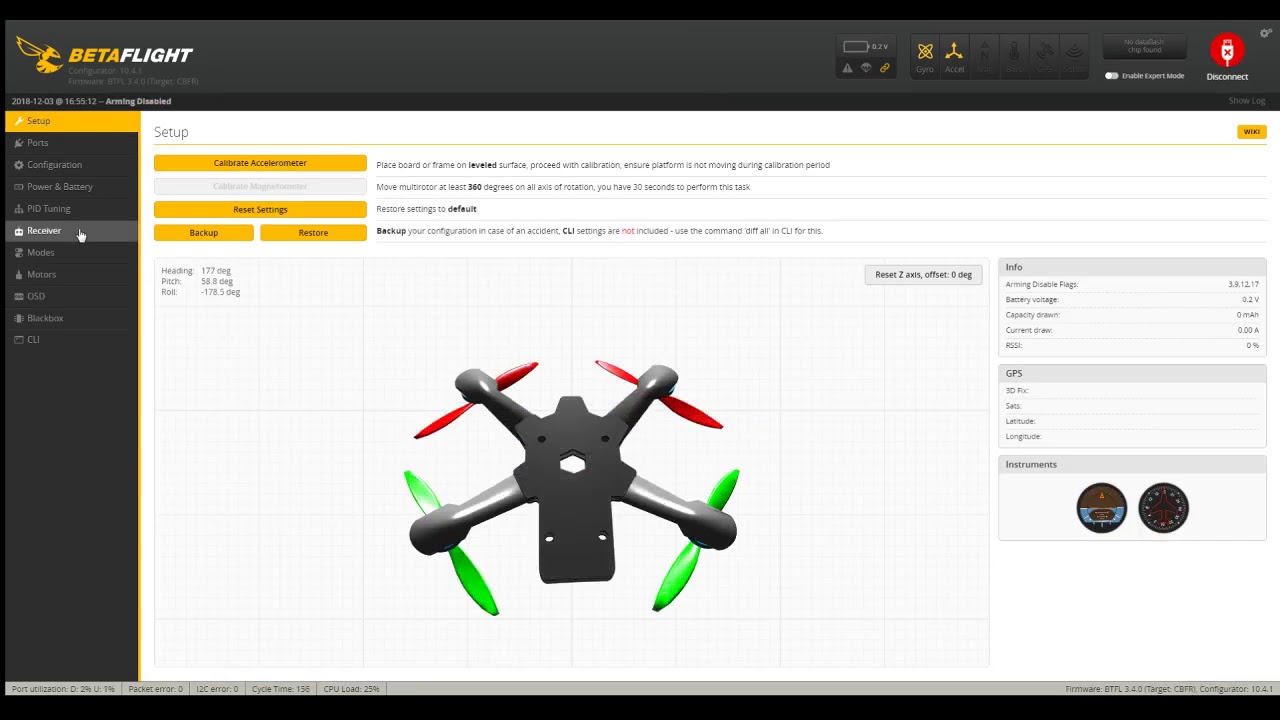The image is a screenshot taken from a website. The background prominently displays the text "BETA FLIGHT," where "BETA" is written in all capital letters in yellow, and "FLIGHT" is in all capital letters in white, both words connected together. Adjacent to the text is a logo depicting a bumblebee with its wings angled backward.

The central part of the image features a detailed diagram, which appears to be an illustration of a drone. The device depicted has a central hub with a hollow center, suggesting it might be mounted onto something. Extending from the central hub are four legs, each ending in a propeller. The two propellers positioned at the top of the image are red, while the two at the bottom are green. 

Above the diagram, there are several clickable buttons labeled "Calibrate Accelerometer," "Reset Settings," and "Backup and Restore." In the lower left-hand corner, there are two circles within a box labeled "Instruments."

This detailed caption effectively captures the visual elements and layout of the screenshot, offering a clear description of the content.